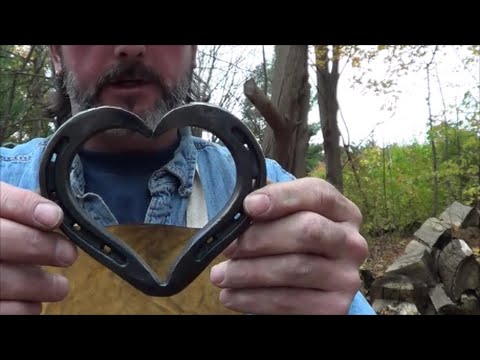In this detailed landscape-oriented photograph, a man is prominently featured holding a heart-shaped horseshoe up to the camera. The horseshoe, originally a standard piece of equine hardware, has been masterfully folded and cut to form a heartfelt shape, showcasing the craftsmanship likely attributed to the man himself. He holds the metal art with both hands, and the details of the horseshoe, including the spots where the nails used to go, are clearly visible.

The man is partially visible, from his torso to just above his nose. His salt-and-pepper beard hints at his age and experience, and he wears a denim button-up shirt over a dark blue t-shirt. To add to his craftsman's appearance, he also dons a leather apron with a white strap around his neck, suggesting he is indeed the blacksmith who created the horseshoe heart.

The background features a lush, green forest, indicative of spring or summer, with thick greenery and trees. To the right of the man, there is a substantial stack of chopped wood, which further implies that he uses fire to heat and shape metal. Above the forest and logs, the upper portion of the image shows a partly cloudy sky.

The photograph is presented in a letterbox format with thick black borders at the top and bottom, focusing the viewer's attention on the detailed craftsmanship of the heart-shaped horseshoe and the stoic presence of the man holding it.